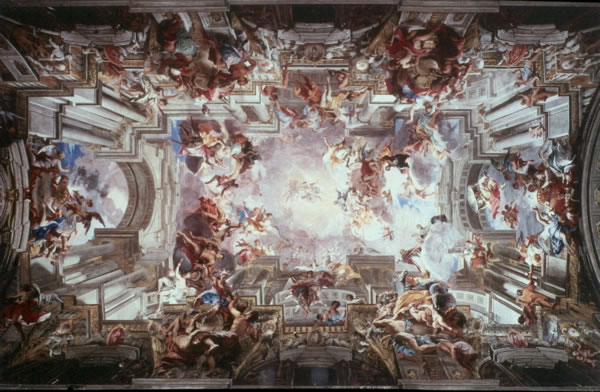The image appears to be an elaborate painting, likely the ceiling of a cathedral or a church, viewed from directly below. The scene is dominated by a bright, cloud-filled sky at its center, with blue patches interspersed with white clouds. Surrounding this central sky are numerous figures clothed in reddish-brown and light blue robes, some of whom seem to be actively engaging with the scene, appearing almost as though they are jumping or floating. Painted columns and arches frame the composition, with characters densely populated around these architectural elements toward the edges of the artwork. The entire painting exudes a sense of movement and divine interaction, reminiscent of old biblical themes, creating a captivating and dynamic visual experience.